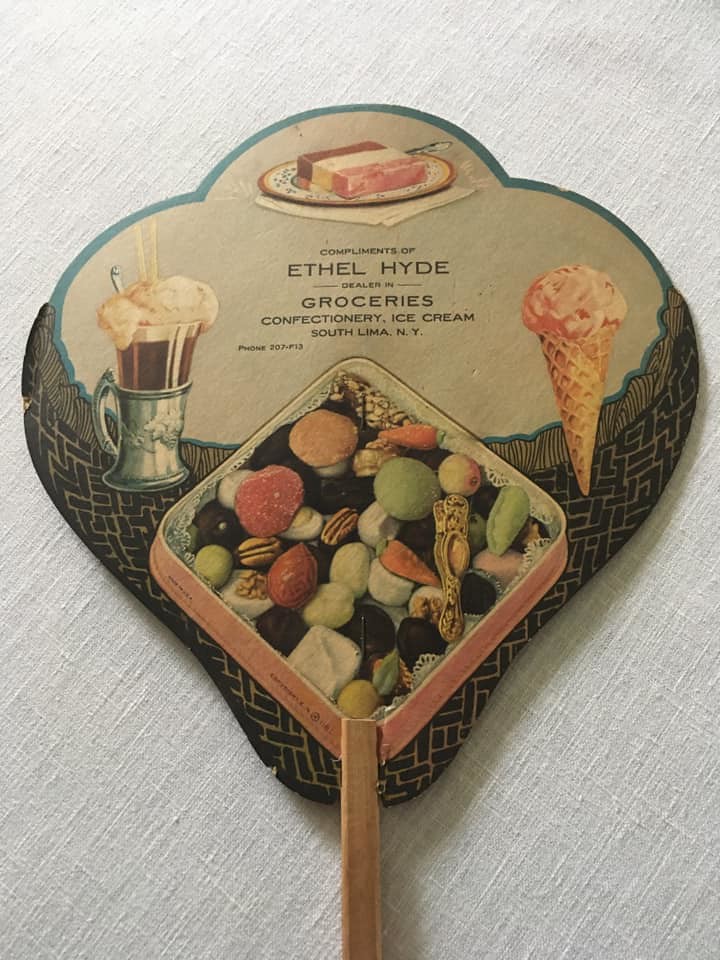This is a detailed image featuring a nostalgic advertisement for Ethel Hyde, a dealer in groceries, confectionery, and ice cream from South Lima, NY. The sign, which is written in a serif font with black text on a gray background, reads: “Compliments of Ethel Hyde, dealer in groceries, confectionery, ice cream, South Lima, NY,” and includes the phone number 207-F13, all held up by a wooden stick. The background is a simple, plain white canvas.

The centerpiece displays a delightful assortment of treats: to the left, there is a fizzing root beer float overflowing with vanilla ice cream in a tin can. At the top, a perfectly plated Neapolitan ice cream showcases its classic chocolate, vanilla, and strawberry layers. To the right, a vibrant pink strawberry ice cream sits charmingly on a waffle cone. Scattered all around the center are various confectioneries, including green candies, pink candies, pecans, and dark chocolates, adding a touch of color and variety to the scene.

Overall, the image has a vintage, possibly hand-drawn design, suggesting it might date back to the 1950s or earlier, creating a charming glimpse into the past.